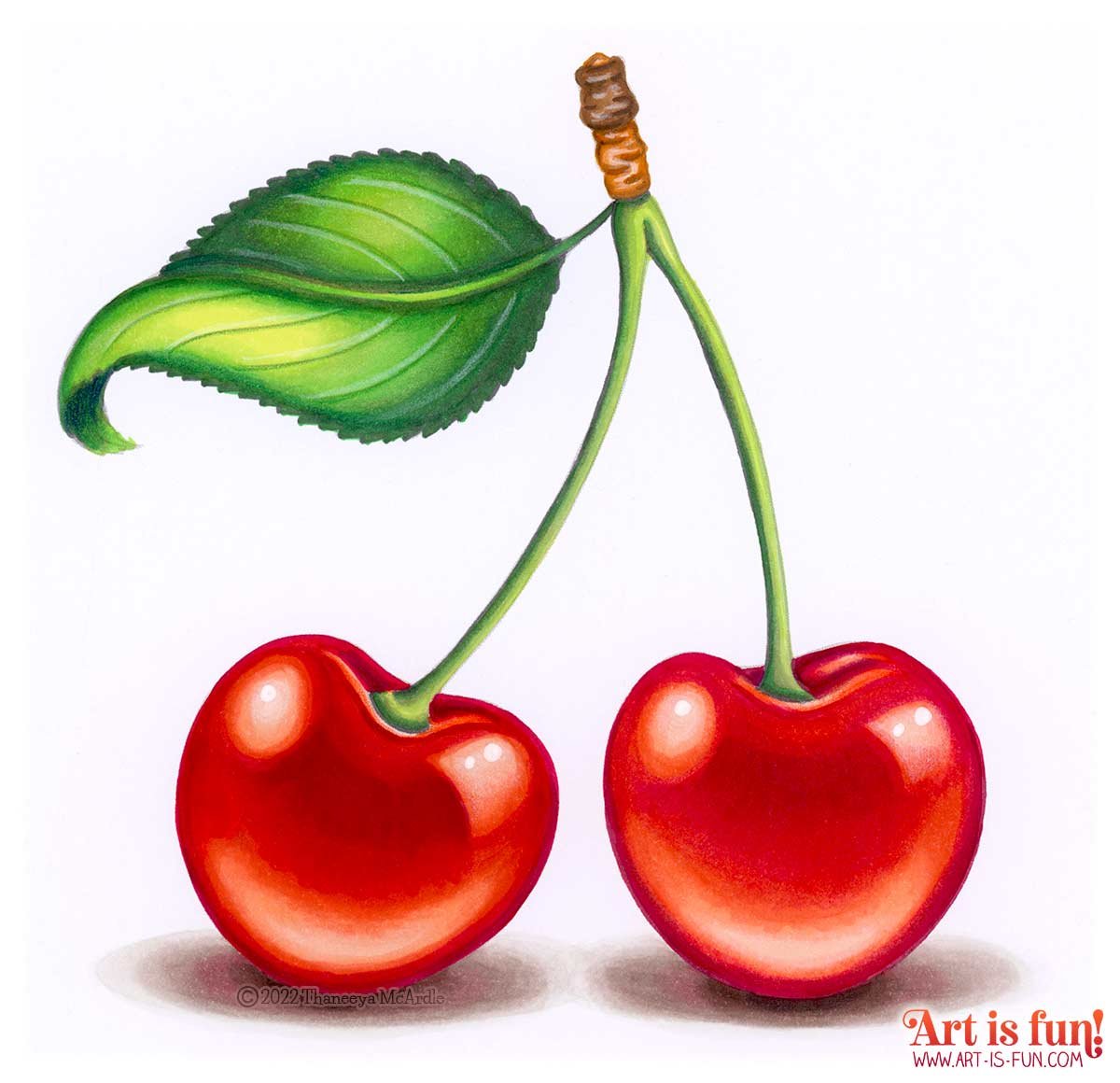This is an illustration, possibly hand-drawn with colored pencils, depicting a pair of vibrant red cherries connected by a V-shaped green stem. At the top of the stem, where it attaches the cherries, there is a darker brown section transitioning into green. The cherries appear fresh and are well-shaded with red tones and touches of white to indicate glares and shadows. On the left side of the cherries, there is a large, slightly curled bright green leaf shaded with green and yellow tones. The cherries cast a subtle shadow beneath them, enhancing the depth of the illustration. In the lower right-hand corner, the text "Art is Fun!" is displayed in an orange-red color, followed by the web address "www.art-is-fun.com" in purple.